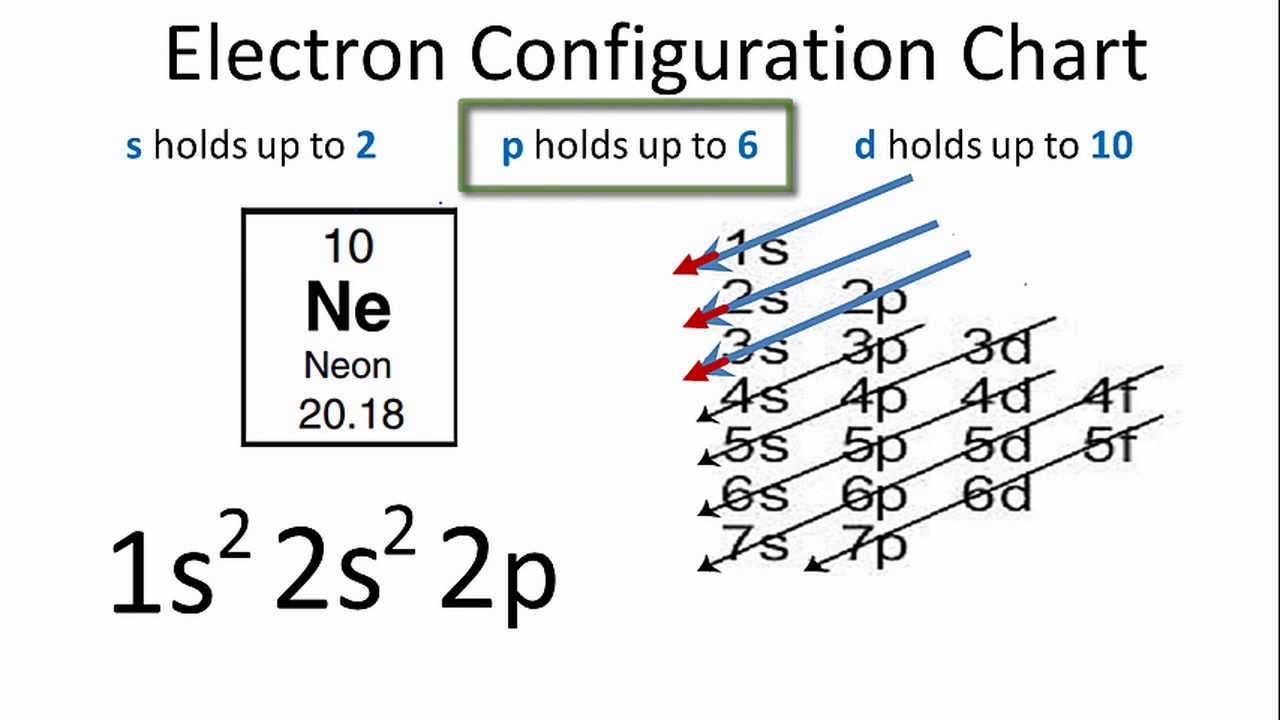The color image features an Electron Configuration Chart prominently displayed on a white background without any borders or frames. At the top, bold black text reads "Electron Configuration Chart." Below this heading, there is a section highlighted by a green box, detailing "S holds up to 2," "P holds up to 6," and "D holds up to 10," with the numbers and letters in blue and the descriptive text in black. To the left of this section is the element Neon, depicted with the periodic table entry featuring the atomic number 10, the symbol "NE," the name "Neon," and the atomic weight listed as 20.18. Beneath this are the electron configuration notations: "1s²," "2s²," and "2p." Towards the bottom right, there are columns labeled from "1s" through "7s," "2p" through "7p," "3d" through "6d," and "4f" to "5f," each accompanied by arrows of various colors. Blue arrows topped with red tips direct towards the configuration, alongside black arrows pointing downwards from "4s" and "3p" to "7s" and "7p." The chart is colored in light olive green, black, blue, red, and white, and provides a comprehensive visualization of electron configurations.